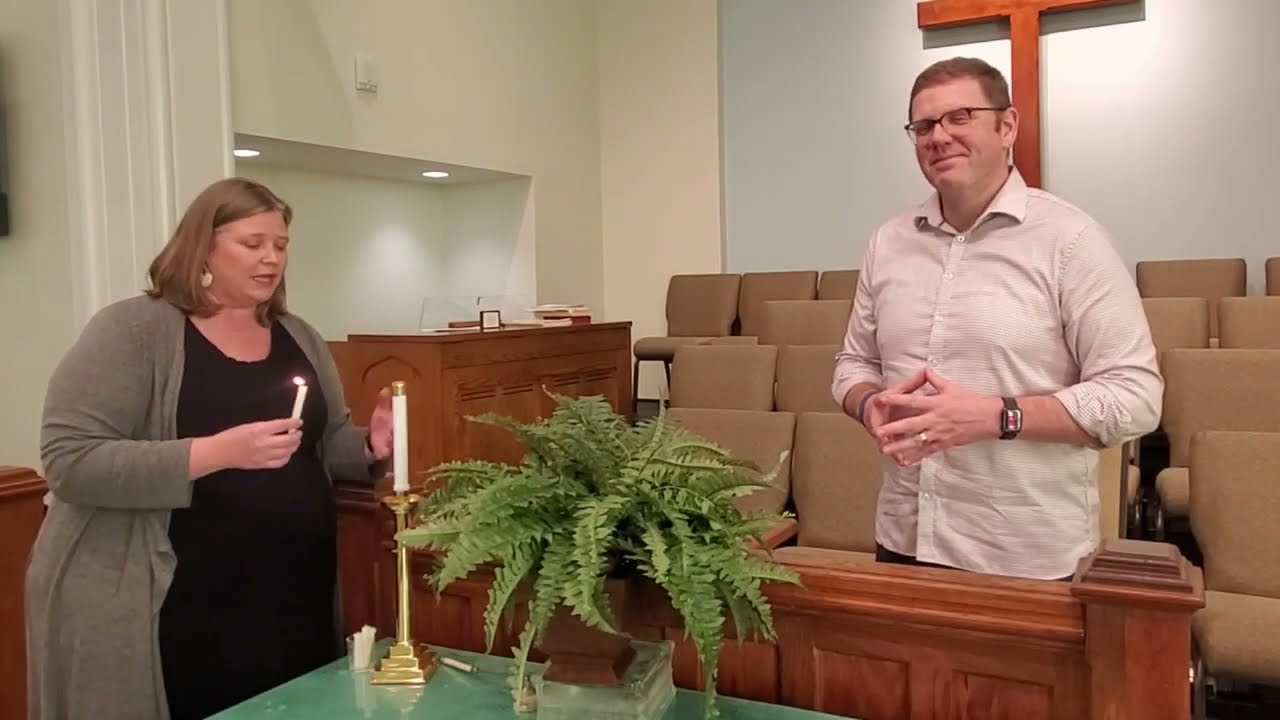In this vertical rectangular photo taken inside a small church, two people stand near an altar. On the left is a heavyset woman dressed in a black dress with a gray cardigan. She has shoulder-length brownish-blonde hair and is wearing earrings. The woman is looking slightly downward and appears to be speaking, her mouth open, as she holds a lit white candle with a brass base in her right hand. In front of her is a green table adorned with a potted fern with long leaves and another candle in a gold holder.

To her right, a man with glasses and short reddish-brown hair stands, facing slightly forward and to his right, with his hands together in front of him. He is wearing a beige collared button-down long sleeve shirt with the sleeves rolled back and a brown wristwatch, and he has a wedding ring on his left hand. Behind him are four rows of brown cushioned chairs, and further back, a light-colored wall can be seen. A large brown cross hangs in the upper right corner of the wall. On the upper left side of the image, a white wall with a cutout possibly leading to another room is visible, along with some spotlights on the ceiling. An organ can be glimpsed to the side, reinforcing the church setting.